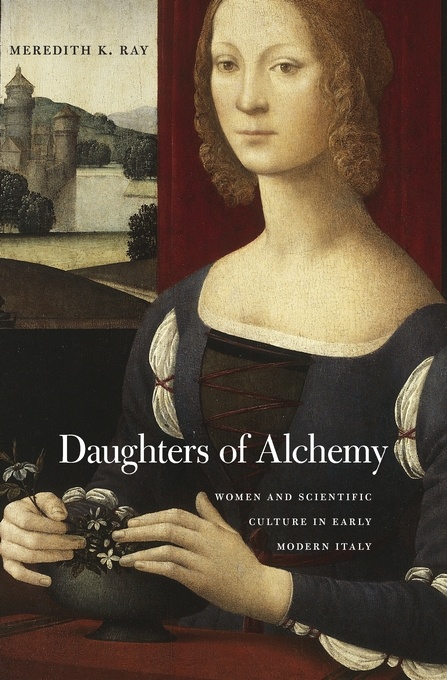This image, likely the cover of a book titled "Daughters of Alchemy: Women in Scientific Culture in Early Modern Italy" by Meredith K. Ray, features a detailed painting of a contemplative young woman from early European or colonial times. The woman, depicted from the chest up, is seated with a dark red curtain as her backdrop. She has short, curly brown hair, partially covered by a bonnet, and is wearing a navy blue long-sleeve dress with a black center and red stitching. Her shoulders are covered, and her neckline dips slightly, revealing the intricate crisscross design of her dress. The woman is gently caressing a bowl filled with white flowers that sits on the table before her. To the left of the woman, an image of a gray-toned, castle-like building with cylindrical towers, mountain ranges, and trees suggests a historical European setting. The author's name, Meredith K. Ray, is displayed at the top in black font. The title of the book is written at the bottom of the image. The overall composition presents a serene and reflective atmosphere, reminiscent of a Florentine painting, with a nod to the Renaissance era.